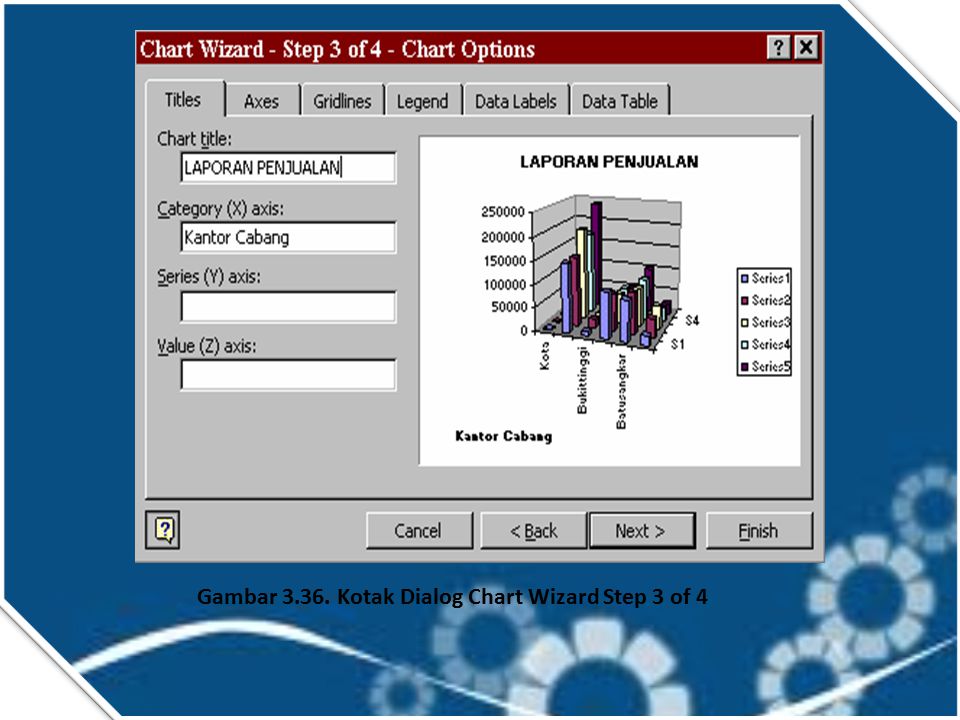The image is a detailed screenshot of a pop-up window commonly seen when creating a chart in Excel or similar software applications. The background of the image is predominantly blue with white circles and a squiggly line towards the bottom. The caption at the bottom of the image reads "GAMBAR 3.36 KOTAK dialog chart wizard step 3 of 4" in black text.

The pop-up window, titled "Chart Wizard Step 3 of 4 - Chart Options," is framed by a maroon strip at the top, featuring a question mark button and a close button (X) at the top right corner. The main area of the pop-up is gray and white, and it is divided into several tabs: Titles, Axes, Gridlines, Legend, Data Labels, and Data Table.

The left column of the pop-up displays labels for different chart components: "Chart Title," "Category (X-axis)," "Series (Y-axis)," and "Value (Z-axis)," although only the "Chart Title" ("Laporin Pendulin") and "Category (X-axis)" fields are populated. The right side of the pop-up features a detailed, colorful 3D bar graph with series labeled 1 through 5, utilizing colors such as yellow, red, and blue. Below the bar graph are action buttons labeled "Cancel," "Back," "Next," and "Finish."